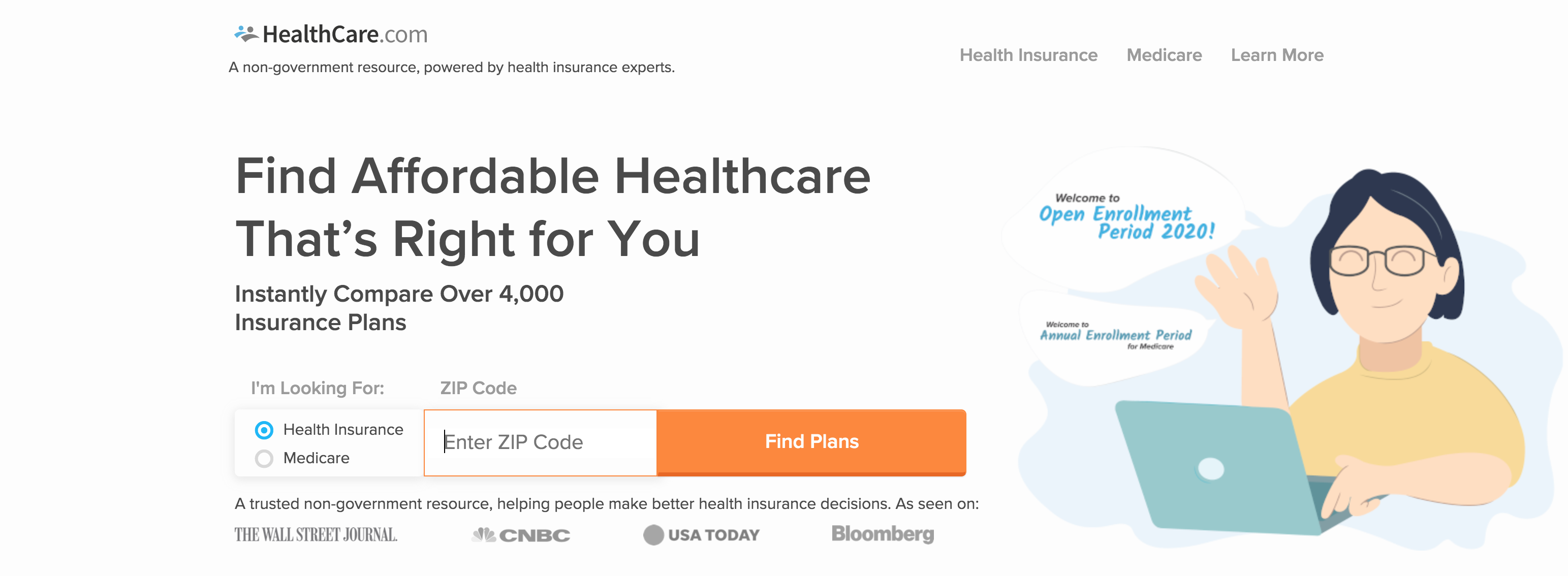**Detailed Caption:**

This is a screenshot of what appears to be a website or a mobile phone screen displayed in landscape mode, making it wider than it is tall. At the top left corner, the website's logo and name, "healthcare.com," are prominently featured, with a small accompanying image to the left of the text. Below the logo, there are small gray letters and a horizontal navigation bar stretching across the screen.

Directly beneath this bar is a bold headline that states, "Find affordable health care that's right for you." Subtext in smaller letters elaborates, "Instantly compare over 4,000 insurance plans." Below this tagline, users are given options to select either "Health Insurance" or "Medicare" from a dropdown menu, alongside a text box to input their zip code. To the right of this input field is an orange button labeled "Find Plans."

Further down, the site showcases logos from reputable sources where it has been featured or advertised, including The Wall Street Journal, CNBC, USA Today, and Bloomberg.

On the right side of the screenshot, there is a stylized, cartoonish illustration of a woman engaging directly with viewers. She is depicted holding a teal laptop, dressed in a yellow T-shirt, and waving her right arm in greeting. She is also wearing black-rimmed glasses. Above her head is a speech bubble announcing the "Open Enrollment Period 2020." Another speech bubble is situated below the first, containing text too small to read clearly.